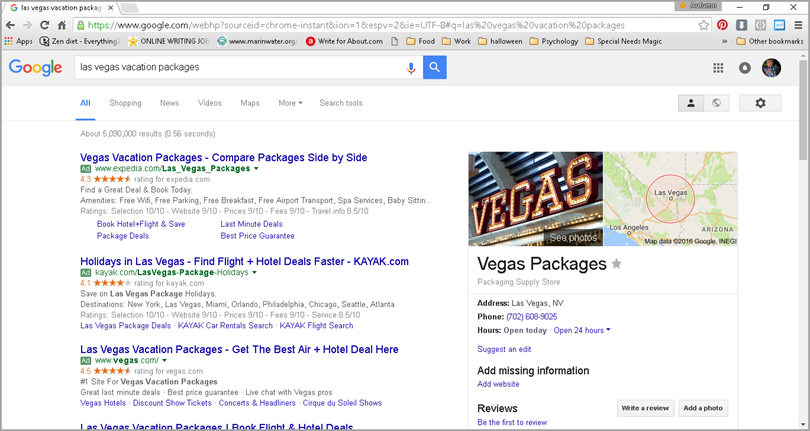The image is a rectangular screenshot with its long side stretching from left to right, depicting a web page viewed in what appears to be the Google Chrome browser, though this is not definitively confirmed. At the very top of the page, there is a search query for "Las Vegas vacation package." The browser interface includes standard navigation icons: a left-pointing arrow, a refresh button, a home button, and a URL bar displaying a lengthy google.com address.

Immediately below the URL bar is the bookmarks bar, featuring shortcuts to various apps including "Zen diet" and others. The main portion of the page shows Google's familiar layout: at the center is the Google logo above a search bar containing the query "Las Vegas vacation packages." The search bar is accompanied by a microphone icon and a blue search button. In the top-right corner, there are icons for a grid menu (likely for Google apps), a notifications bell, and a circular user icon indicating the logged-in user.

Beneath the search bar, navigation options are listed, including "All," "Shopping," "News," "Videos," "Maps," and "More," along with search tools. The "All" option is highlighted in blue and underlined, showing it is the active tab. Following this, there are three paid advertisement links, each highlighted in blue text. The first ad reads "Vacation Vegas vacation packages compare packages side by side."

On the right-hand side of the page, a map of Las Vegas is displayed, alongside a related image labeled "Vegas."